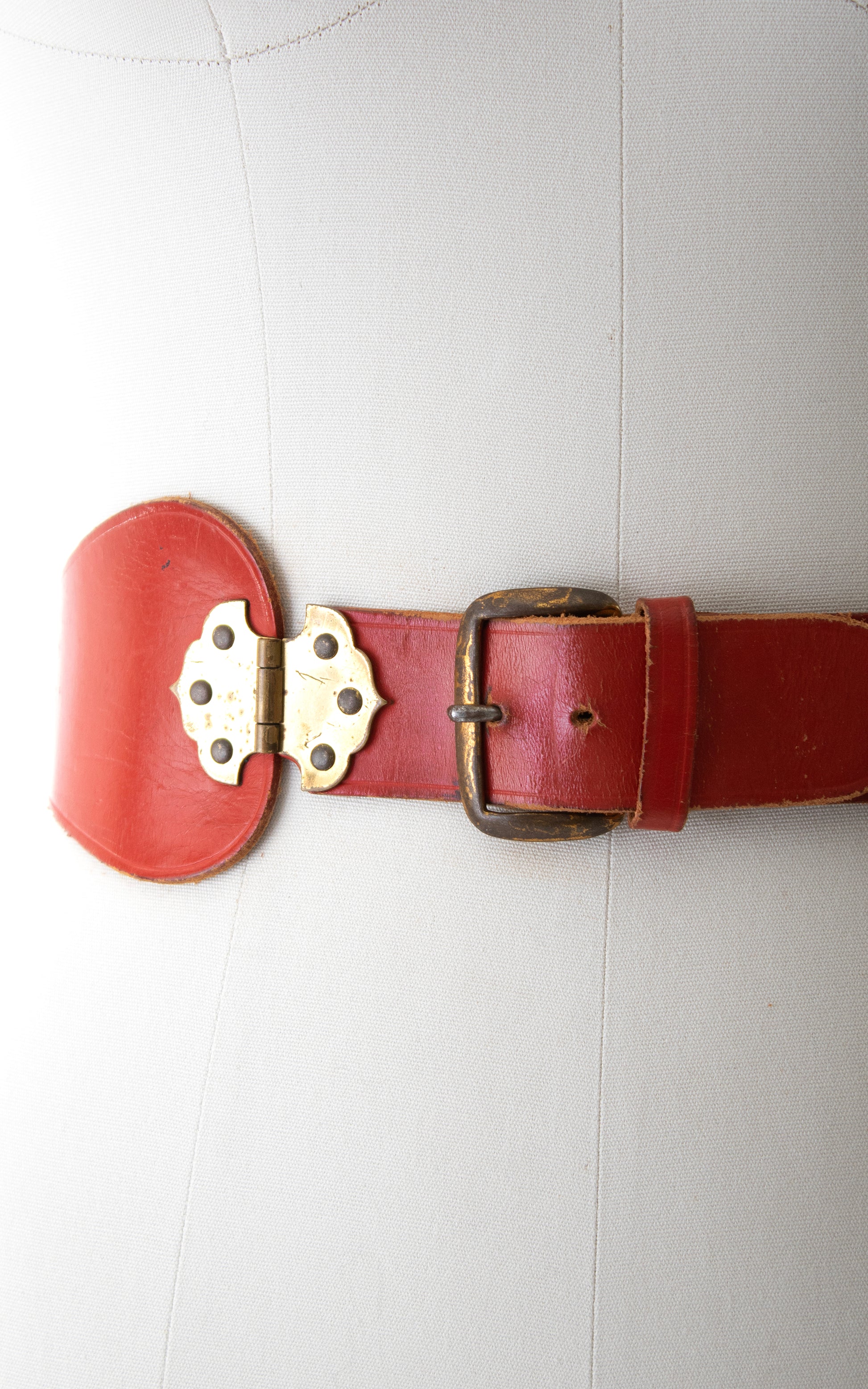The vertically aligned rectangular photo has a background that transitions from white on the left to a lighter gray on the right, resembling a coarse, canvassy or plastic material with vertical lines. The image frames a worn red leather belt that extends nearly the full width from right to left, wrapping around what appears to be a dress form or mannequin torso. The belt features a heavily rusted buckle, which once may have been gold, now displaying a mottled mix of gold and brown. Adjacent to the left of the buckle, there's a metal piece holding two sections of the belt together, adorned with three small screws, retaining its gold hue. The belt noticeably shows signs of age with stretched holes and frayed edges, adding to the sense of wear and vintage charm. The dress form itself is light cream, tapering inward at the waist, contributing to the overall subtly elegant composition of the image.